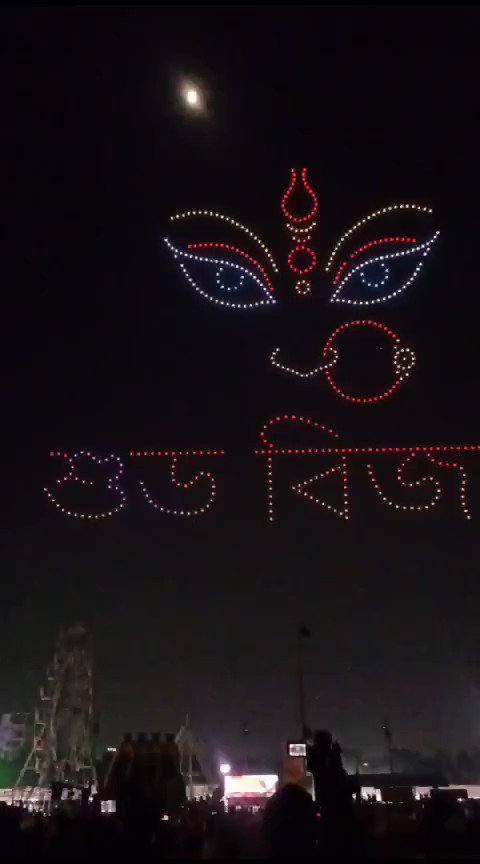The photo, taken at night during what appears to be a festival or at an amusement park, captures a dazzling light show against a dark sky. The main attraction is a formation created by numerous colorful lights, likely drones or fireworks, forming the image of a face. The face features striking blue eyes, yellow eyebrows, and a yellow nose adorned with a prominent red nose ring. Below this vivid display, text in a foreign language adds to the mystique. To the left of the image, there is a discernible Ferris wheel, while at the bottom, the silhouettes of an audience gaze upwards in awe. The lower part of the image also depicts small building structures, possibly shops, with one slightly taller than the rest. Above the captivating face formation, the moon shines brightly, enhancing the enchanting, festive atmosphere. The array of lights includes red, purple, yellow, green, blue, and white, demonstrating an impressive range of colors.